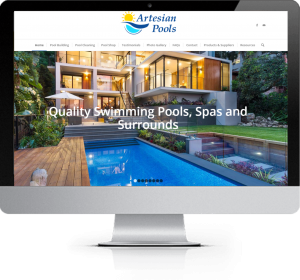The image depicts a website displayed on a Mac monitor. The monitor features a black frame on the left, top, and right sides, with a silver bottom edge and a matching silver stand. The website itself has a white border at the top. The website's header features a centered yellow sun with navy blue and sky blue waves beneath it, and to the right, the text "Artesian Pools" is written in navy blue.

Below the header, there is black text accompanied by navigation tabs, although the text is too small and blurry to discern. Further down on the website, there is an image of a modern home characterized by numerous large glass windows framed in white. To the right of the house, there is a small patch of green grass and brick stairs. On the left, there is a deck-like area. The central focus of the image is a blue swimming pool. The caption under the pool image reads, "Quality swimming pools, spas, and surrounds."